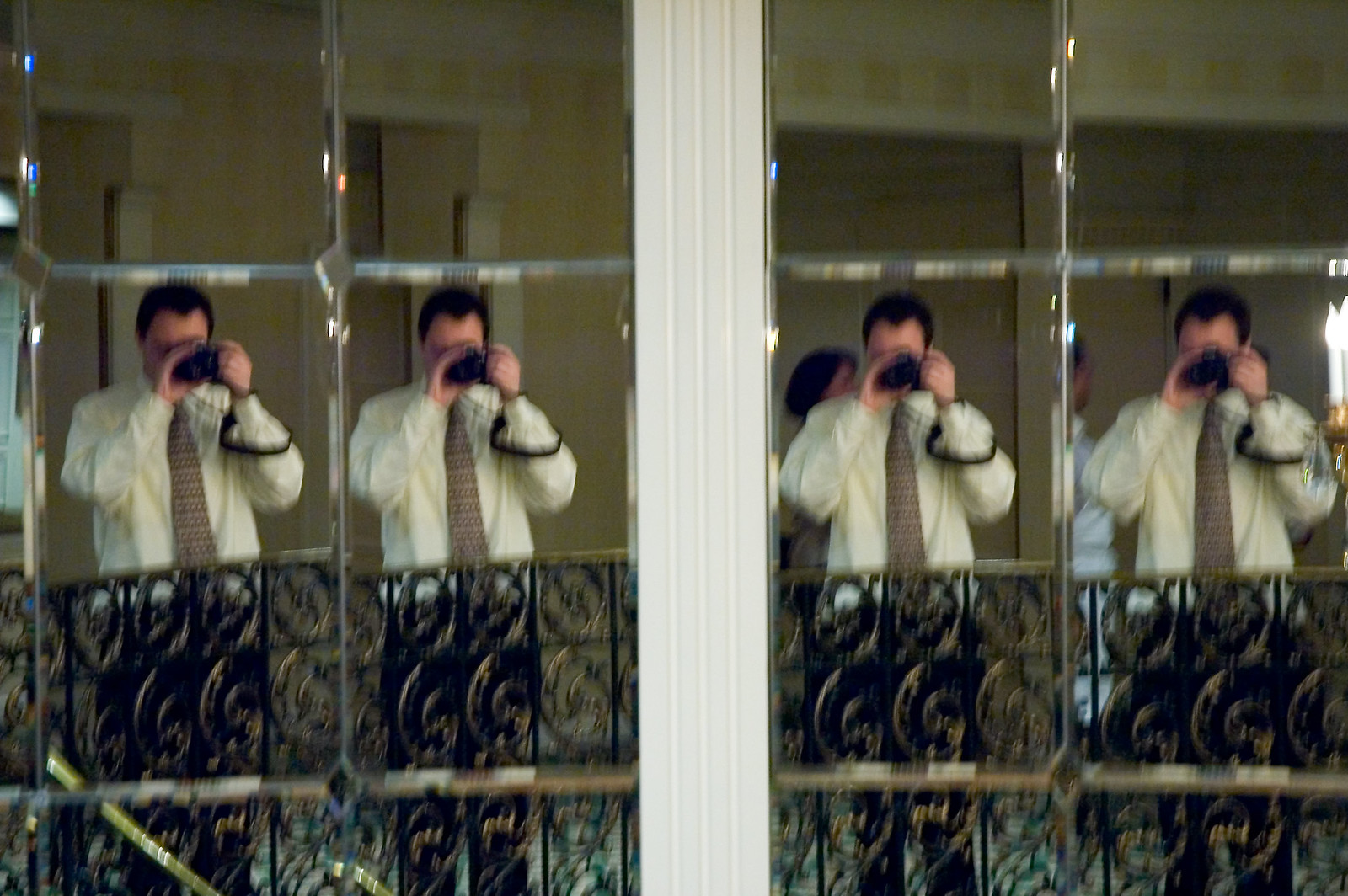This photograph captures a man with black hair, characterized by a widow’s peak, standing on an indoor balcony and taking a picture of his reflection in a paneled mirrored wall. The mirrored wall reflects his image four times. He is dressed in a white long-sleeve button-up shirt and a brown necktie, accessorized with a brown wristwatch on his right hand. He's holding a black camera, with the strap visible around his left wrist. Behind him, a wrought iron balustrade with intricate brass paisley designs runs along the edge of the balcony. Additionally, there are glimpses of a woman and a man in the reflections on the left side, suggestive of this being inside a hotel room with a door visible in the background.